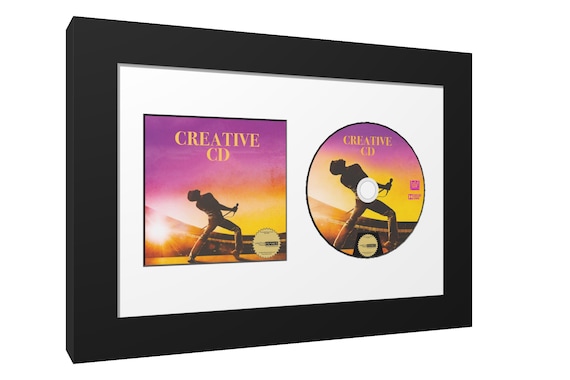Displayed against a clean, white background is a three-dimensional, black wooden frame with two cutouts, showcasing a “Creative CD” album. On the left side of the frame, a square cutout houses the CD cover, which features bold yellow text reading "Creative CD" amidst a vibrant palette of pink, yellow, and violet with an image of Freddie Mercury iconic from the Live Aid performance, energetically arching his back and holding a microphone. On the right side, a circular cutout holds the CD itself. The entire presentation is encased in what appears to be a glass cover, maintaining an organized and visually appealing display. The detailed and colorful artwork stands out sharply against the stark white background, highlighting the framed, commemorative essence of the CD and its cover.